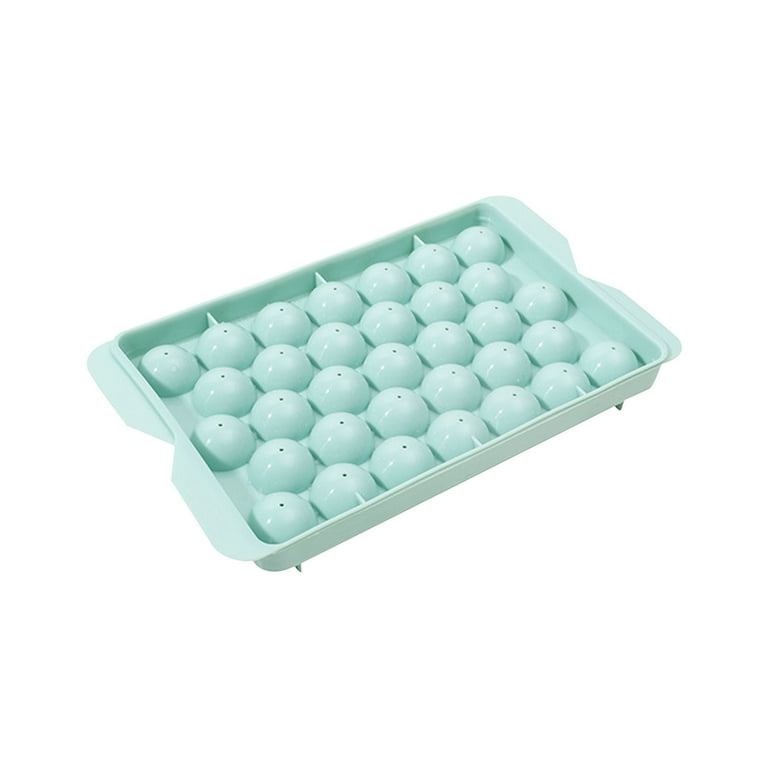In this photograph, there's a turquoise blue, or perhaps light green, ice cube tray, prominently centered against a stark white background. The ice cube tray, which appears to be made of a flexible rubber material with plastic elements, is notably turned upside down, displaying a series of evenly spaced, round-bottomed molds designed to produce spherical ice cubes. Each mold features a small hole, presumably for air to escape and to facilitate easy release of the ice. This innovative tray also includes small legs or feet, suggesting it could be used in this inverted position, possibly indicating that the visible part might serve as a lid for the water-filled tray beneath. The tray is capable of making dozens of spherical ice cubes at once, making it practical for various cooling needs. Its neat arrangement and vibrant color make it an eye-catching product, likely found on retail platforms such as Amazon, catered towards buyers looking for unique kitchen accessories or even molds for candy or cake decorations.